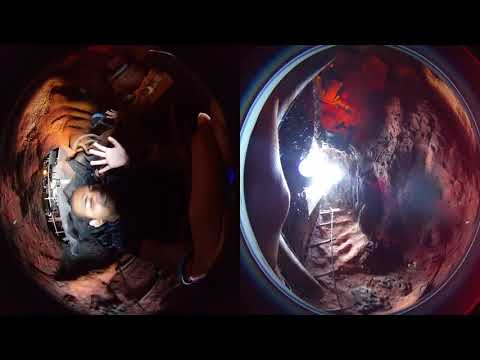In the image, two side-by-side circular frames, resembling fishbowl lenses, capture a scene inside a dark rock cavern. The left frame features a man with olive skin, wearing a black shirt, smiling, and waving at the camera with his palm facing out. He appears to be blocking a light source, whose glare illuminates his face and hand. The surrounding environment is rocky, with visible trails and dirt, creating a semi-creepy, underground tunnel atmosphere. The right frame offers a look further down the cavern, showcasing more rock walls and a railing, with sunlight filtering in, giving it a slightly brighter yet still eerie ambiance. Both images are tilted 90 degrees, contributing to the disorienting feel of the scene.